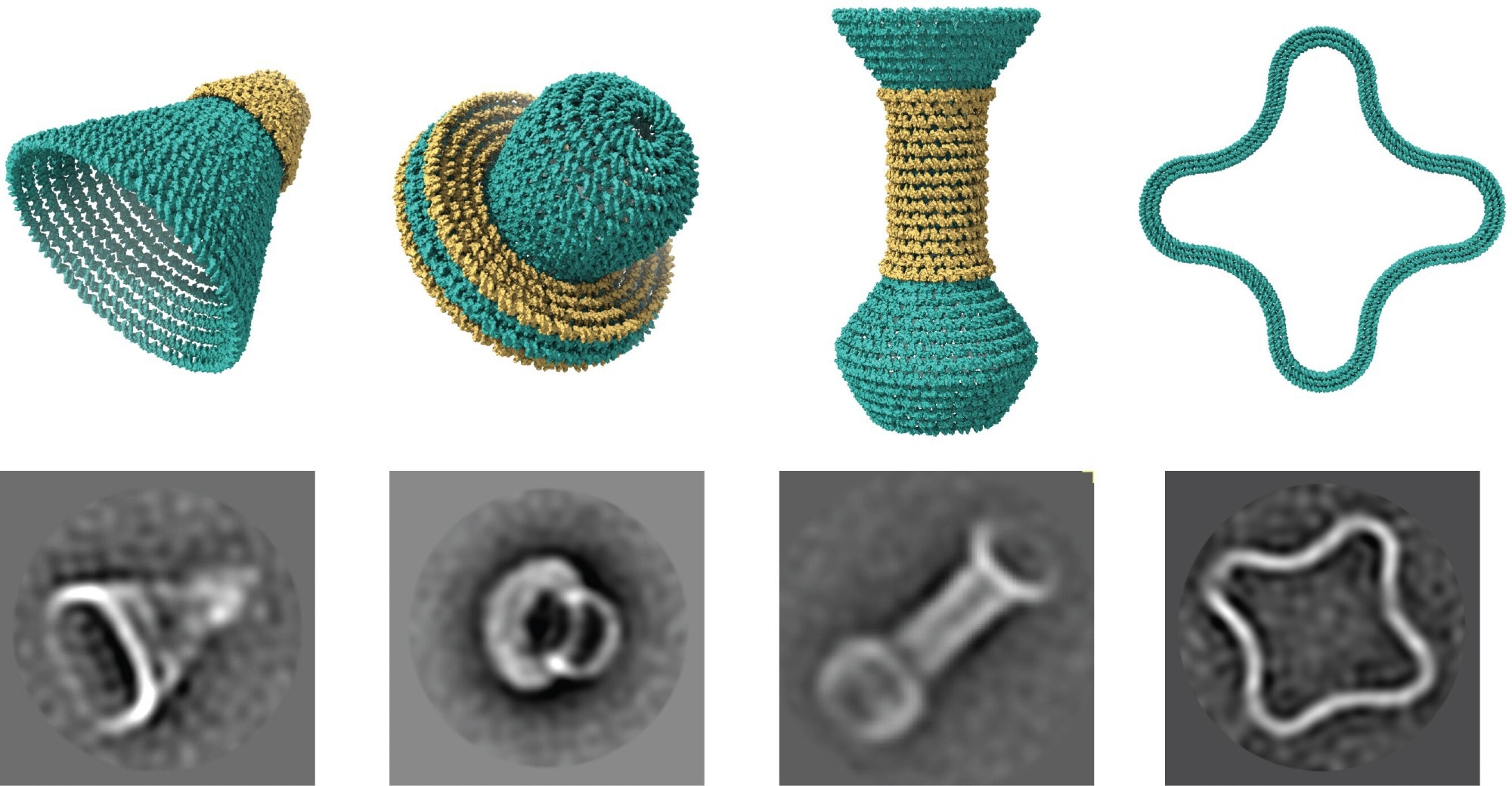This image, resembling a diagram from a textbook or scientific paper, is organized into two rows on a white background. The top row features four colored, artist-rendered shapes: the leftmost is a teal bulb shape with a golden base resembling a shuttlecock, the next is a golden green pacifier-like structure with a large teal plume on top, followed by a dome-shaped object with a gold middle section and a diamond-shaped teal base, and finally, a teal circular cross shape. The bottom row contains corresponding black and white images of these objects, as they might appear under a microscope. Each grayscale image mirrors the shape above it, with textures and outlines defined in white, offering a detailed, realistic view contrasting with the colorful artistic renderings above.